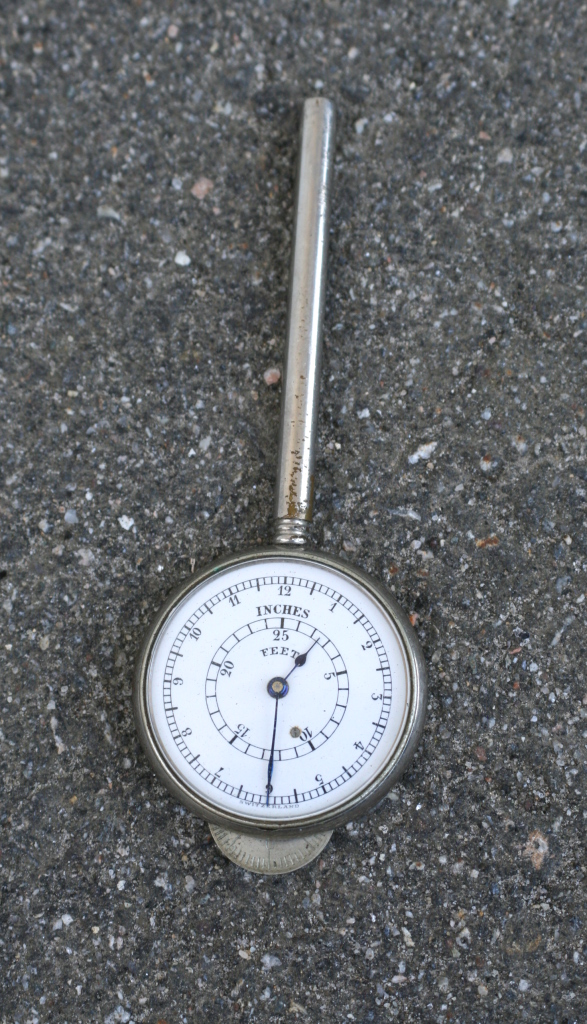This image features a well-worn depth counter, primarily silver in color. The device resembles a traditional pocket watch with a long, tarnished silver stem extending from its top. The circular face of the counter has a white background, meticulously marked with detailed measurements. 

The outer ring of the face is calibrated in inches, displaying numbers from 1 to 12, with finer millimeter increments between each inch. The inner circle is dedicated to feet, marked at intervals of 5, 10, 15, 20, and culminating at 25 feet, with individual foot markers between these major divisions.

Beneath the main dial, a silver half-circle extension is appended to the device, featuring engraved hash marks. The engravings are directly etched into the metal, contrasting the drawn measurements on the primary face.

The depth counter rests on a rough, black asphalt surface, interspersed with small, protruding stones in brown and white hues. The device's silver components, especially the pole connected to the circular face, exhibit signs of tarnishing, indicating age and usage.